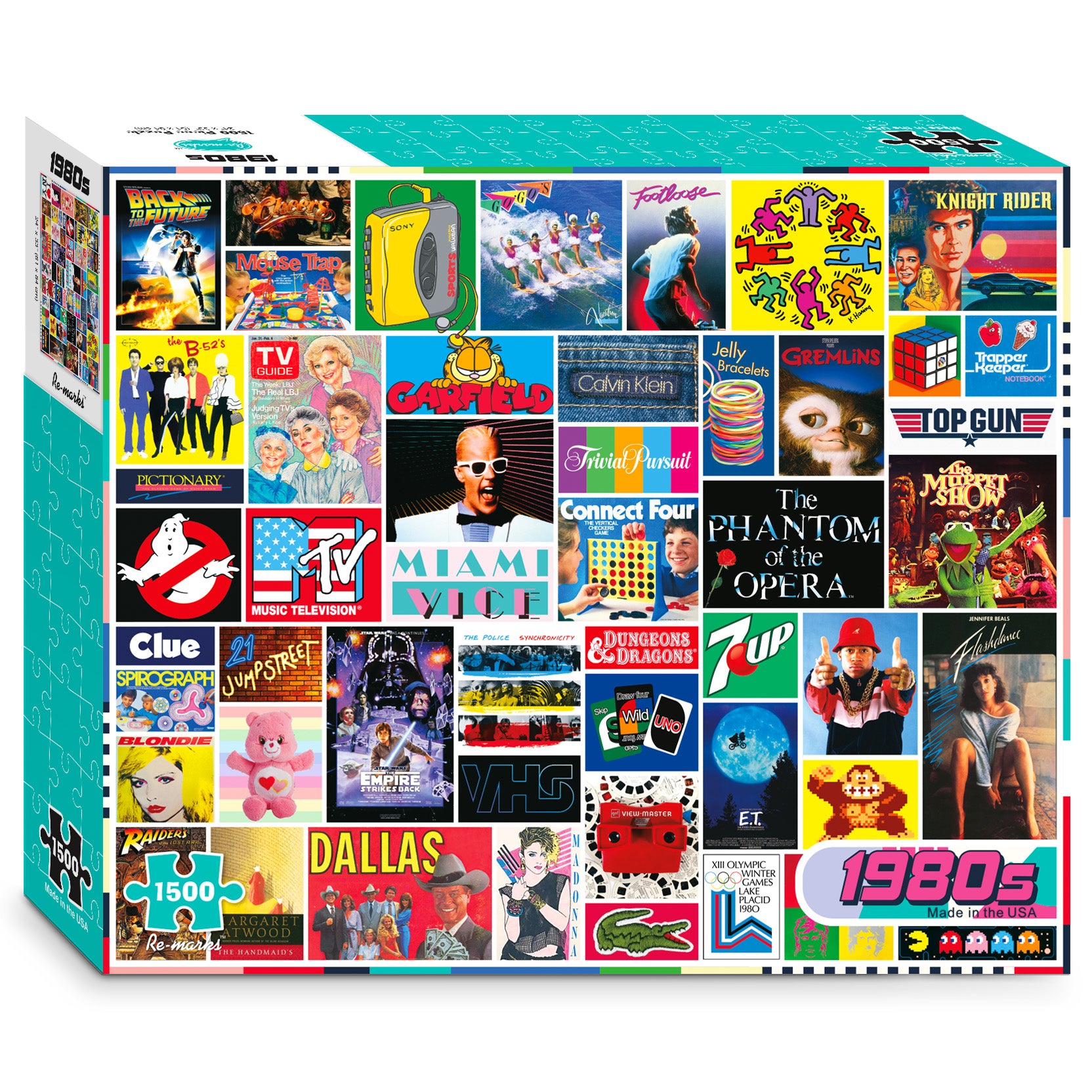The image depicts a puzzle box set against a bright white background. The front face of the box is adorned with a collection of images from movies, video games, and other pop culture references. These images are divided into small, square or rectangular segments, showcasing various types of art, people, and text. Prominently, in the bottom right corner of the box, there is a 'Pac-Man and ghost' graphic with the text "1980s" boldly highlighted in pink. Additionally, the box's sides are a teal aqua color, featuring printed puzzle piece shapes, and there are distinguishing black puzzle pieces on the top and right sides, indicating the set contains 1500 pieces. The overall presentation, including the number '1500' written again on the bottom left within a teal puzzle piece, confirms this as a puzzle box. The intricate design and the specific details such as the era "1980s" add to its nostalgic appeal.